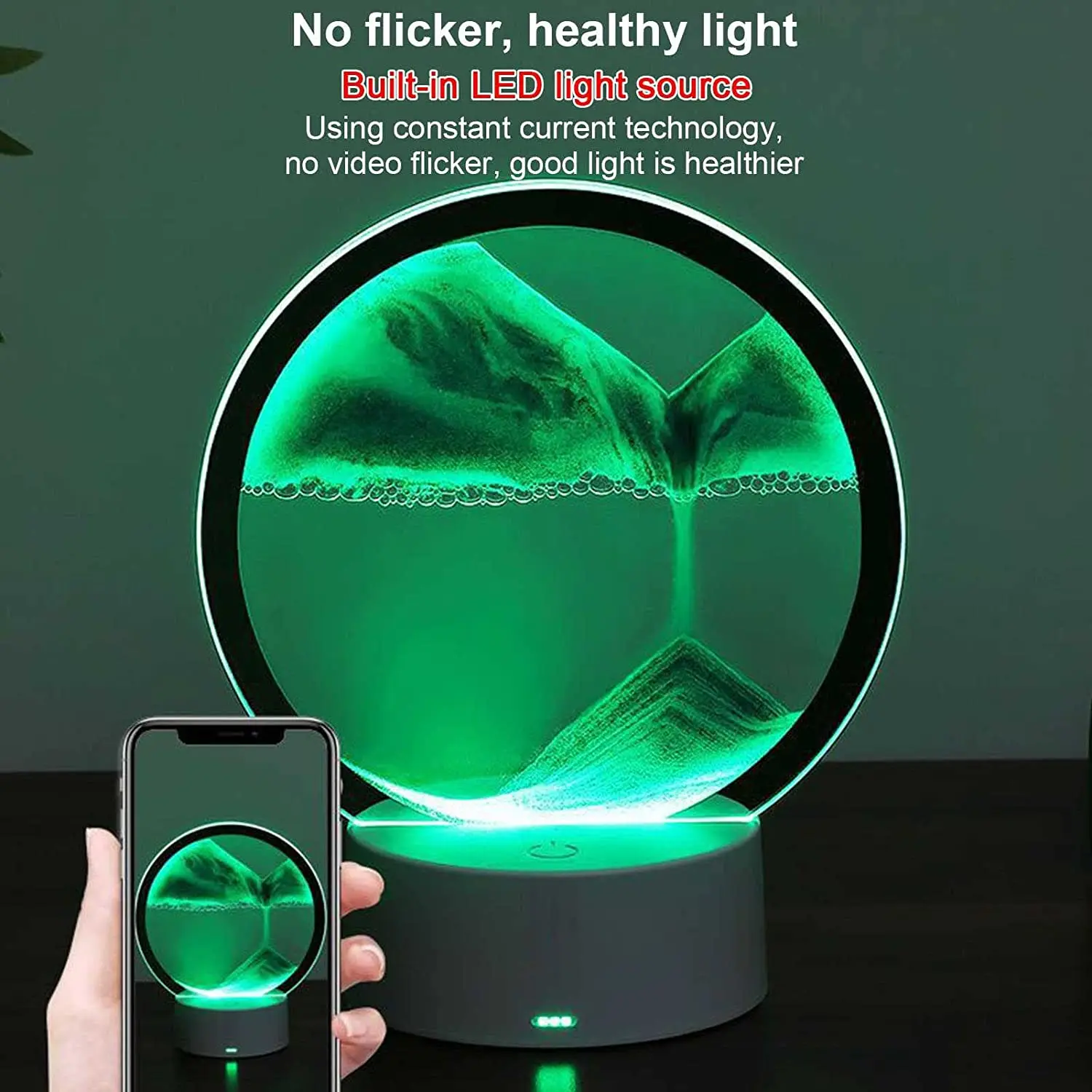The poster advertises a built-in LED light source with the headline "No Flicker, Healthy Light." It highlights the product’s use of constant current technology to ensure no video flicker, promoting healthier lighting. Central to the image is a bright circular LED screen lamp featuring a power button and a base with an illuminated power indicator. The background of the image is dark green, enhancing the prominence of the featured product. Intricate design elements include a green swirl with bubbles and what resembles a whale tail, alongside stacked washcloths at the bottom, creating an artistic and engaging visual appeal. Additionally, in the lower left corner, there is a hand holding a smartphone displaying a duplicate of this advertisement, underscoring the message that no flicker and healthy light are central to the product’s benefits.